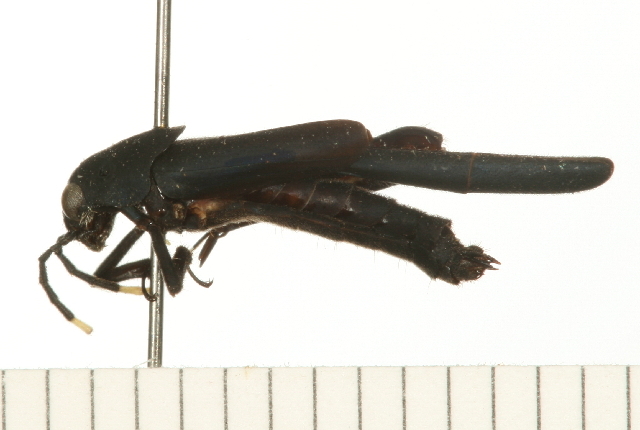The photograph depicts what appears to be a dark-colored insect, possibly a grasshopper or locust, that has been impaled on a metal pin, suggesting it is a specimen for entomological study. The insect's body, which varies in color from dark black with lighter brown spots to a dark brown with a tinge of green, is positioned in profile with the head on the left side of the image and the body extending to the right. The insect features two prominent antennae that are dark with cream-colored tips, a large dark eye, and what appear to be long wings along its cylindrical body. The metal pin securing the insect is attached to a vertically striped cream and brown platform that likely serves as a measurement label. The image's background is a solid white, emphasizing the insect and its details against a clean, minimalistic backdrop.